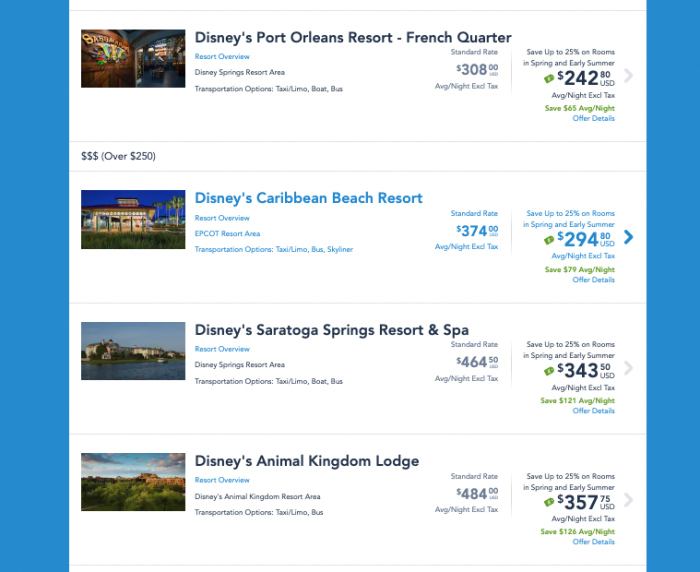This webpage showcases a selection of Disney resorts, complete with pricing and clickable overviews. The first resort featured is Disney's Port Orleans Resort – French Quarter, neatly enclosed between two blue bars. It is presented with a detailed rate comparison; the original rate of $308 is marked down to a bold price of $242 for tonight. A clickable resort overview link is available for additional information.

Next is Disney's Caribbean Beach Resort, listed with an original rate of $374, now offered at $294. This section includes a resort overview, along with links to Epcot and transportation options, and highlights the moderate price range with $3 signs.

The third listing is Disney's Saratoga Springs Resort and Spa, originally priced at $464 but currently available for $343. As with the previous listings, a resort overview is accessible, offering more details about inclusions and amenities.

Lastly, Disney's Animal Kingdom Lodge is showcased, featuring an initial rate of $484 now reduced to $357.75. A clickable resort overview is provided for further exploration of the resort’s features and offerings.